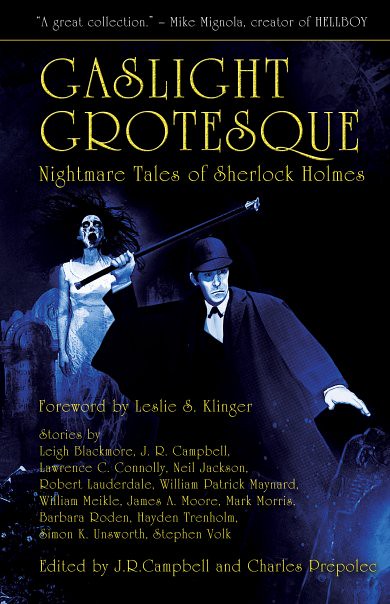The poster is titled "Gaslight Grotesque: Nightmare Tales of Sherlock Holmes" set against a stark black background. At the top, in white text, the words "A Great Collection" are prominently displayed, followed by the mention of Ivan Mike Magluler as the co-curator of Hellboy. Below, the subtitle "Gaslight Grotesque: Nightmare Tales of Sherlock Holmes" introduces the collection with a thin yellow line separating the sections of text. There's a foreword by Leslie S. Klinger and includes stories by various authors such as Lee Blackmore, J.R. Campbell, Lauren C. Connolly, Neil Jackson, Robert Lauderdale, William Polnyk Maynard, Jessica A. Moore, Mark Morris, and more. 

The central illustration is a striking black and white drawing. On the left, a female ghost with long, disheveled black hair and a white dress, her bloodstained face frozen in a scream, adds a chilling presence. On the right, a man resembling Sherlock Holmes is dressed in a dark suit and cape, with a white shirt and his iconic cap. He holds up a long staff in his right hand, with the head of the cane visible over his shoulder. The drawing exudes an eerie and haunting atmosphere. At the bottom, the poster notes that the volume is edited by J.R. Campbell and Charles Prepost, using a loopy handwritten font. This detailed artwork and comprehensive information emphasize the collection's spooky and mysterious theme.